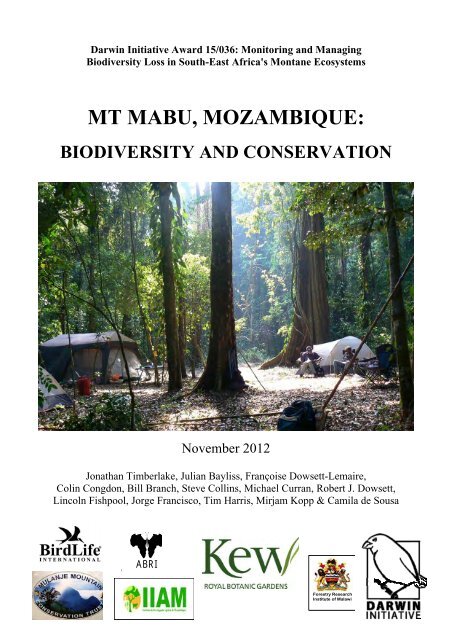The poster showcases a campsite set in the lush forests of Mount Mabu, Mozambique, centered around the theme of biodiversity and conservation. Dated November 2012, the image highlights a collaborative effort involving various organizations such as BirdLife International, ABRI, IIAM, Kew (Royal Botanic Gardens), and the Darwin Initiative, as indicated by their logos at the bottom. The scene features several tents, including a gray, white, and blue one, nestled among towering redwood trees with dense green foliage. Campers are seen sitting in fold-out chairs amidst a ground covered with dead leaves, emphasizing the untouched natural beauty of the area. At the top of the poster, bold text reads, "Darwin Initiative Award 15-036: Monitoring and Managing Biodiversity Loss in Southeast Africa's Montane Ecosystems." The overall ambiance is accentuated by bright sunlight filtering through the tree canopy, hinting at the pristine and serene environment being preserved and studied.